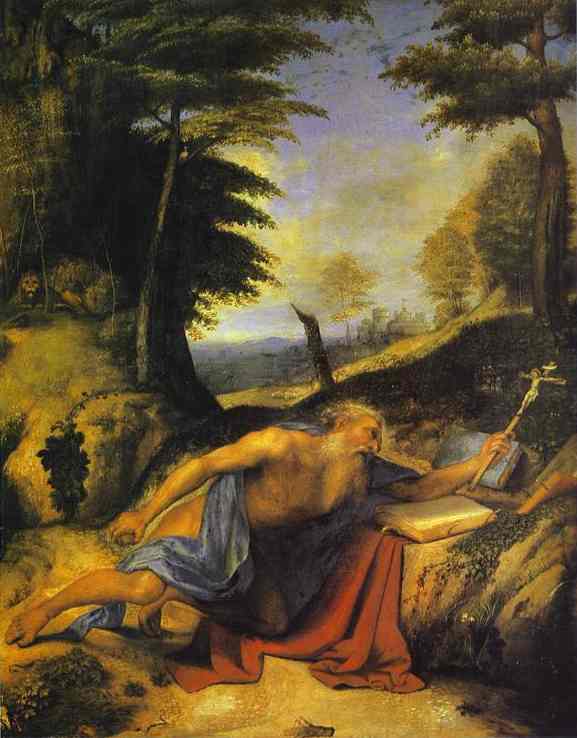The oil painting depicts an elderly Christian saint in a natural, woodsy outdoor setting, under a bright, clear blue sky. The figure, who has short white hair and a long white beard, is draped in a loose blue and red robe and appears to be in a state of anguish or contemplation. He is reclining against a rock formation, partially falling over onto an elevated piece of land. In his left hand, he holds a tall crucifix featuring a miniature depiction of the crucifixion of Jesus. An open book lies beside him on a red cloth, and another large blue book is propped up against the knoll he's leaning on. The background includes a detailed landscape of trees, hills, a gray area, and some distant buildings, with the soil beneath him being a yellowish light brown. The natural lighting in the painting is bright and emphasizes the serene yet poignant atmosphere.